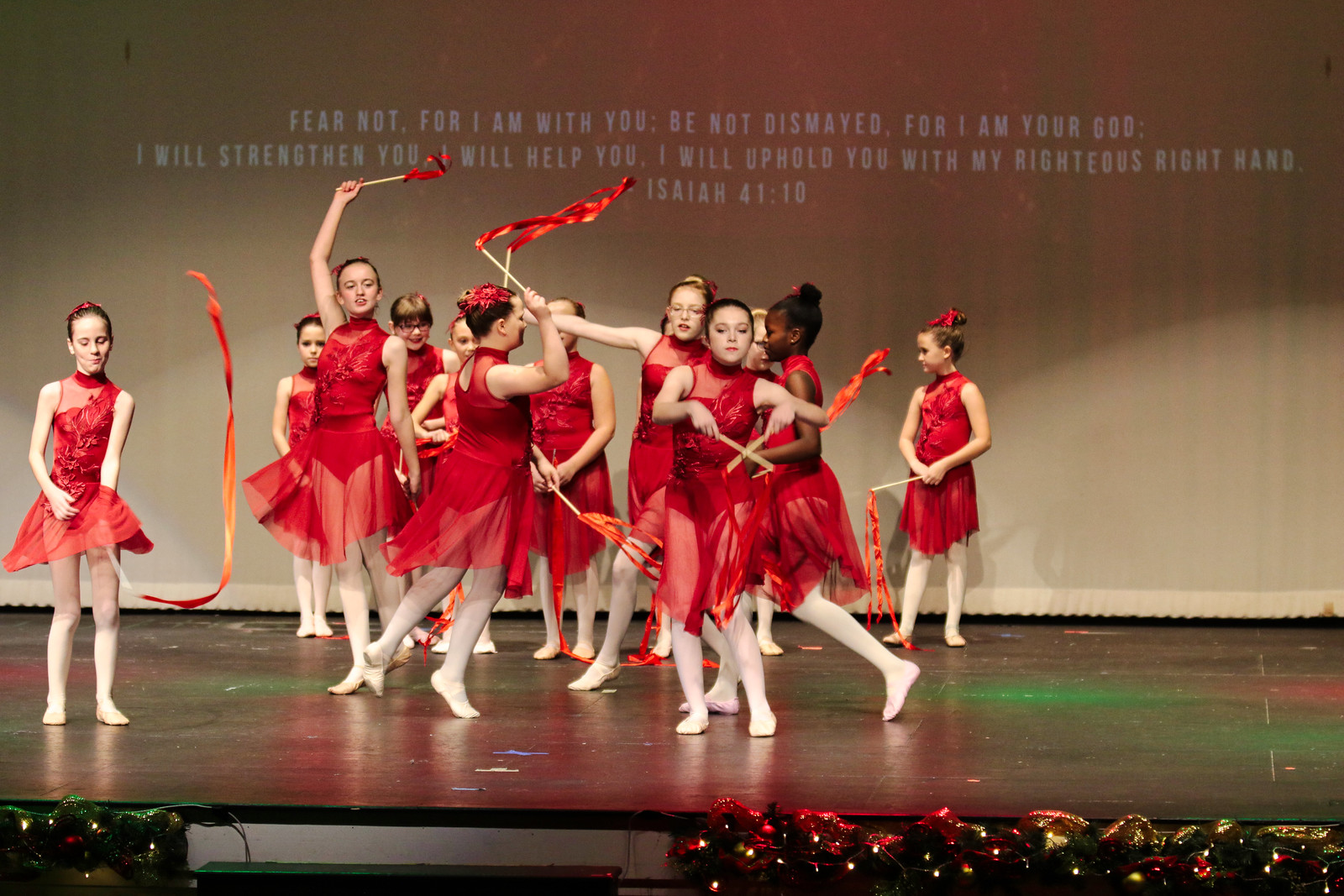In this horizontally aligned photograph, a dozen young teenage girls are performing on a stage adorned with Christmas decorations and illuminated by colorful spotlight reflections of green and pink. The stage itself is a dark gray color, contrasting with the girls who are wearing red dresses with lacy bottoms, white tights, and white dance shoes. Their hair is styled in updos, and they energetically wave red glittery streamers attached to sticks above their heads, reminiscent of rhythmic gymnastics. Behind them, a wall displays the text: “Fear not, for I am with you. Be not dismayed, for I am your God. I will strengthen you. I will help you. I will uphold you with my righteous right hand. Isaiah 41:10.”